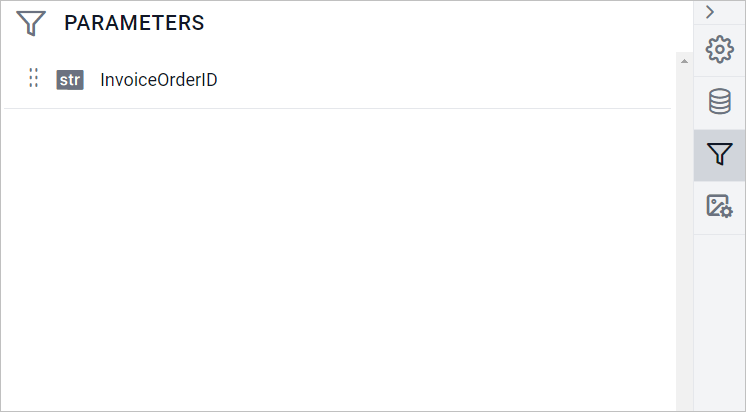In this image, the web page or menu depicted appears largely empty, giving an impression that it may not be fully loaded or it is intentionally designed with minimal content. Dominating the screen is a vast expanse of white, creating a stark and uncluttered background. At the very top, the word "Parameters" is prominently displayed in bold black text. Just below this heading, in a smaller font, is the text "123 Invoice ID."

Towards the upper right corner of the interface, there are several small, clickable icons. One icon resembles a gear, likely indicating an access point for an options menu. Beneath the gear, there are additional icons—one may represent an image, possibly for adjusting brightness or other visual settings. The remainder of the screen is predominantly blank, emphasizing the minimalist aesthetic or incomplete content.

At the very bottom of the page, the phrase "Edit Layout" is inscribed in small blue font, possibly offering a customization option. Anchored at the extreme bottom is a blue clickable button featuring a plus sign and the text "New Parameter," suggesting functionality to add new parameters or items to the web page or menu.